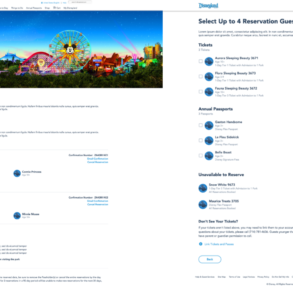This screenshot captures the Disneyland package booking page, albeit in a minimized and somewhat blurry state. The top-left corner features an image that includes a Ferris wheel with Mickey Mouse in the center, encircled by various amusement park rides. Beneath the image, there are two lines of text, followed by two reservations listed under different names, each accompanied by an icon—a blue circle with a dark blue Mickey Mouse head in the center. To the right of these reservations are the names of the party members.

On the right side of the screenshot, "Disneyland" is prominently displayed at the top. Just below it, instructions prompt users to "Select up to four reservations," though the text is partially cut off. Underneath, there is a section for tickets, showing three different ticket options, none of which are selected. Following this is a category for annual passports, listing three different options, again, none of which are chosen. Near the bottom, under "Unavailable to Reserve," two additional options are shown, indicating items that cannot be booked.